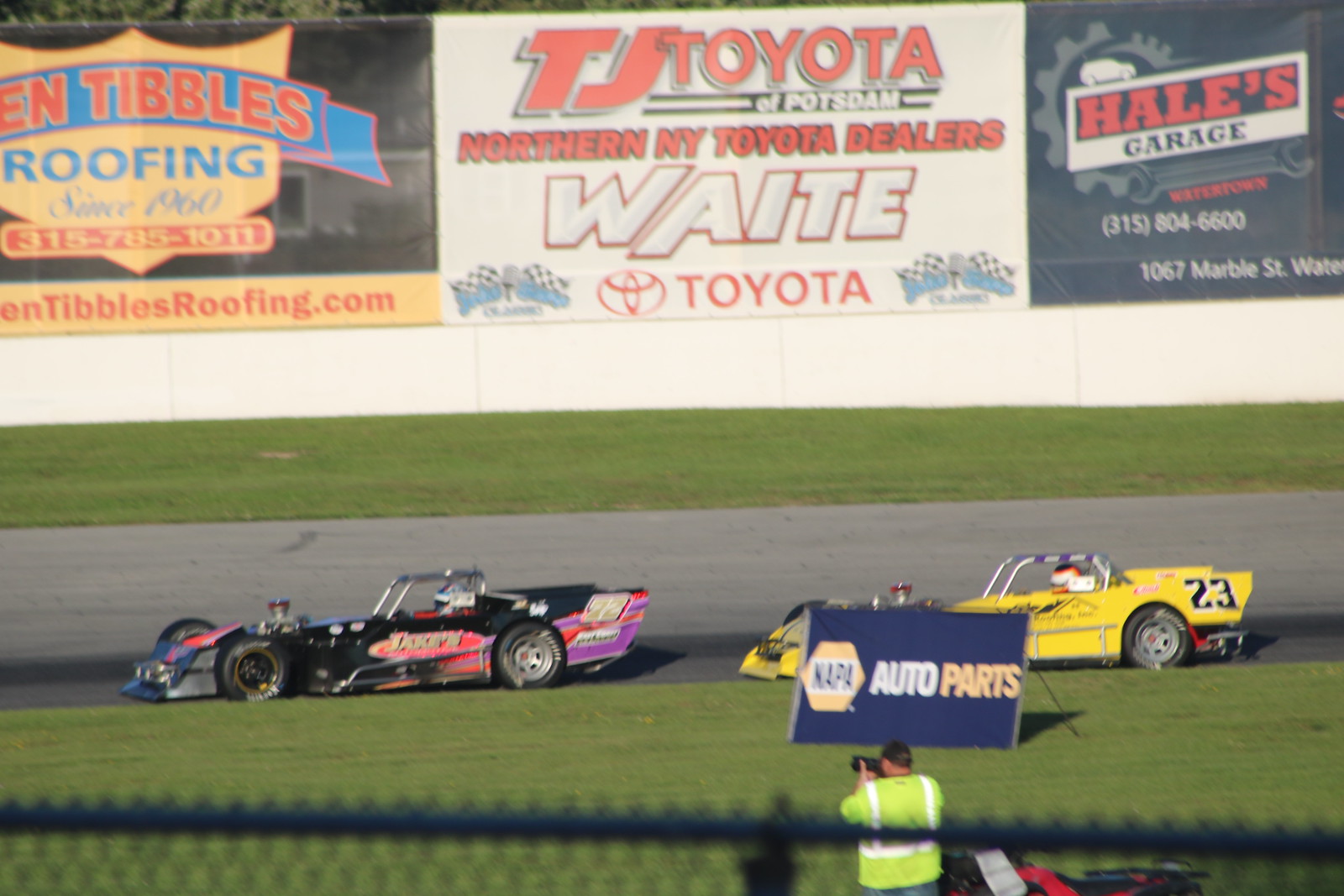The image depicts a vibrant racing scene featuring two race cars on a gray, paved track that diagonally tilts upwards from the middle left towards the right. The track is bordered by lush, green grassy areas above and below. Dominating the horizon is a white barrier festooned with large billboards.

In the foreground, a heavy-set man in a yellow and white shirt, blue jeans, and a safety vest holds a black camera, partially obscured by a blue or gray fence. To his side, a red and black four-wheeler sits on the grassy expanse. The track hosts two race cars: a black car with the number 22 and "Jake's" emblazoned in yellow and pink on the side, and a yellow car with a blue number 23. Near the yellow 23 car, a blue and yellow Napa Auto Parts sign stakes its claim.

High above the track, three billboards prominently display their ads. The leftmost sign advertises Ian Tibbles Roofing, established in 1960, all presented on a yellow and red background. Centrally, another advert conveys "TJ Toyota, Northern NY Toyota Dealers" in striking red letters, surrounding white text that says "Wait" and "Toyota." The final billboard on the right heralds Hales Garage with black and white text on a red backdrop, including their contact information and partial address in Watertown, NY. 

This detailed tableau captures the intensity and sponsor-laden atmosphere indicative of a lively race in Watertown, New York.